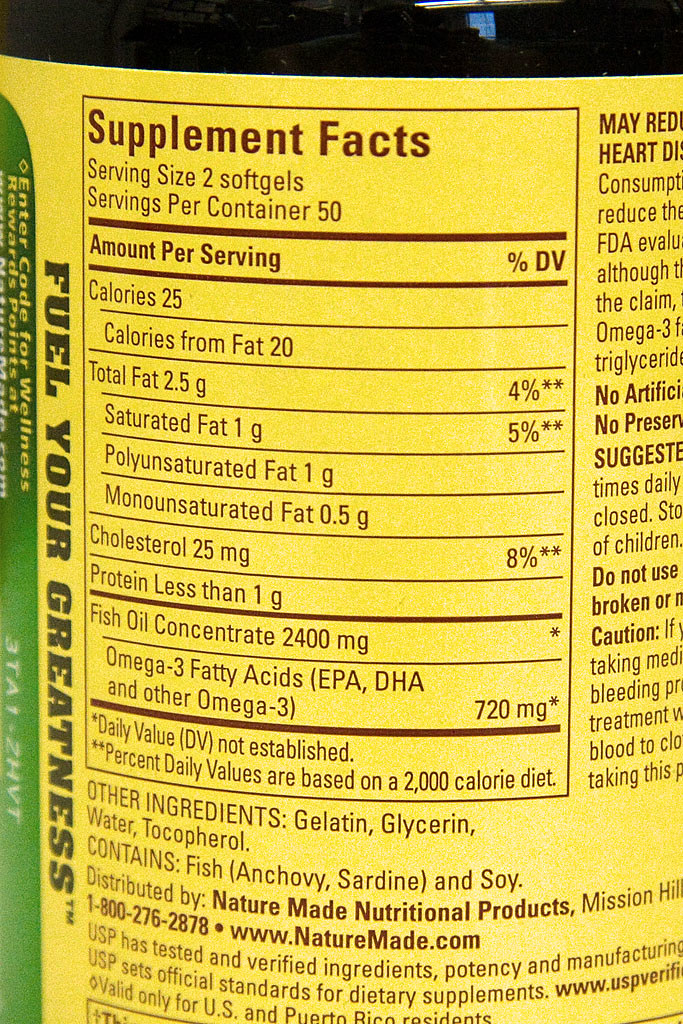This close-up image features the side of a Nature Made vitamin container, predominantly yellow in color with some green bordering on the left side. The text, primarily in thin brown font, details the supplement facts which start with "Fuel your greatness" in dark black letters. Below this, it specifies a serving size of two soft gels with 50 servings per container. Nutritional information includes 25 calories per serving, with 20 calories from fat, 2.5 grams of total fat, 1 gram of saturated fat, 1 gram of polyunsaturated fat, and 0.5 grams of monounsaturated fat. Additionally, it lists 25 milligrams of cholesterol, less than 1 gram of protein, 2,400 milligrams of fish oil concentrate, and 720 milligrams of omega-3 fatty acids (comprising EPA, DHA, and other omega-3s). The other ingredients are gelatin, glycerin, water, and tocopherol, and it contains fish (anchovy, sardine) and soy. This product is distributed by Nature Made Nutritional Products, with contact information provided as 1-800-276-2878 and www.naturemade.com. The label also indicates that the ingredients, potency, and manufacturing have been tested and verified by USP, which sets official standards for dietary supplements. The top section of the product seems to have a black, smooth reflective surface, likely made of glass or plastic.